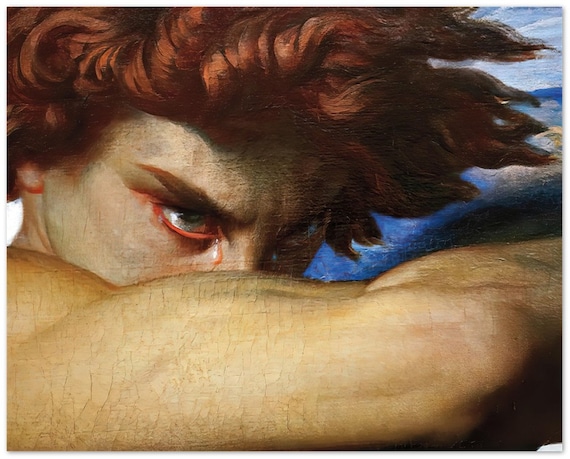This painting features a light-skinned individual with a distinctly sinister appearance. Dominating the foreground is their arm, partially obscuring their face in a mysterious manner. The person's eyes are particularly striking, displaying unsettling, red-tinged hues reminiscent of salmon, with off-white pupils that enhance their eerie gaze. Their short, flowing hair and eyebrows are vivid shades of red, and their brows are furrowed menacingly. The individual's nose is subtly concealed behind their arm, adding to the overall enigmatic and foreboding aura. Behind them, a background of blue, gray, and white tones provides a stark contrast, further emphasizing the dark shadows cast near their elbow. The composition and color choices evoke a deeply sinister atmosphere.